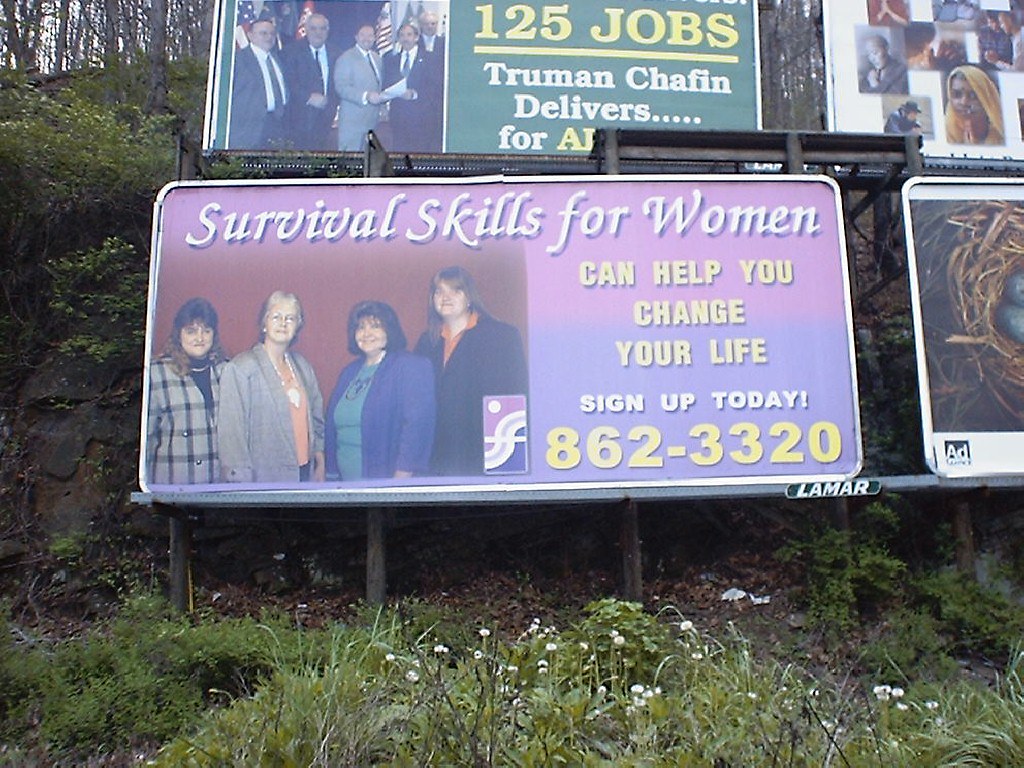This outdoor daytime photograph, taken along a rural roadside, depicts a cluster of four billboards mounted against a slightly overgrown grassy area with unmanaged clover patches and dandelion stalks. These billboards are positioned in front of a small rock-faced wall that appears to be part of a hill or mountain, with barren trees extending into the distance, suggesting the scene may be set in late autumn or winter. The focus of the image is on the billboard in the lower left corner, which features a bold purple background and white text at the top that reads "Survival Skills for Women." Below the text, there is a photograph of four middle-aged Caucasian women, each with 80s-style perms and wearing blazers, suggesting they offer empowerment or training programs. On the right half of the billboard, yellow text proclaims, "Can help you change your life. Sign up today," followed by a contact number, 862-3320. Although partially visible are another billboard above it, hinting at a political message, and another with an image of bird eggs in a nest, their content is less discernible.